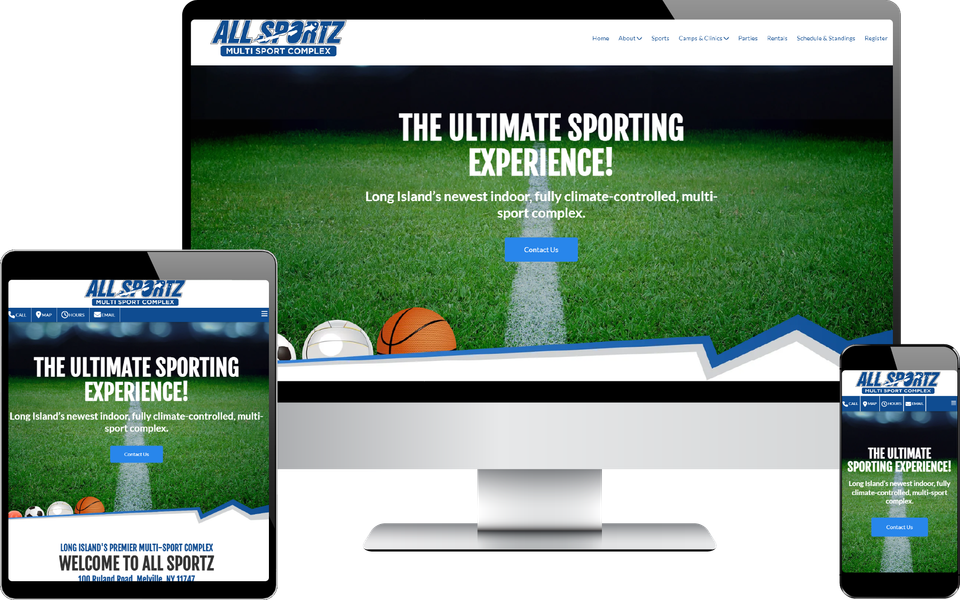This photo illustration depicts different versions of the All Sports Multi-Sport Complex website as viewed on a computer screen, tablet, and mobile phone. 

On the computer screen, the website is shown with navigation links located from the middle to the right side of the display. Though the text is slightly challenging to read due to its distance, identifiable links include those for "Sports," "Parties," and "Register." Below the links, an image of a football field is visible, complete with green grass and a white painted line dividing the field. Above the field, a bold statement reads, "The Ultimate Sporting Experience: Long Island's Newest Indoor Fully Climate-Controlled Multi-Sport Complex." Beneath this, a blue rectangle with white lettering prompts users with "Contact Us." The bottom of the computer screen showcases an image featuring a soccer ball, volleyball, and basketball, along with an illustrated mountain adorned in white, gray, and blue layers.

The tablet version of the website maintains a similar layout but with slight differences. Links are grouped within a horizontal blue bar situated underneath the title of the complex. The tablet also includes the mountain illustration with text in the white area reading "Welcome to All Sports."

The mobile phone version, designed for a smaller display, presents a streamlined view. It retains the essential links but forgoes the mountain illustration to fit the compact screen size.

Overall, this detailed illustration effectively showcases the versatile, user-friendly design of the All Sports Multi-Sport Complex website across multiple devices.